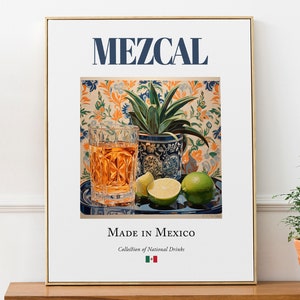This vertical rectangular photograph features a piece of artwork displayed either on a brown wooden shelf or potentially on the floor against a white wall with a baseboard visible. The artwork is encased in a thin brown or gold frame and prominently displays the word "Mezcal" in big blue letters at the top and "Made in Mexico" in smaller black letters below a colorful central image. This image depicts a drink, possibly mezcal, in a glass filled with a light brown liquid, accompanied by sliced limes and a full lime on a silver plate. A plant or pineapple appears in the background against a vibrant wallpaper with blue and yellow designs. There is additional text at the bottom, likely referencing a collaboration, but it is too small to read clearly. On the right edge of the photograph, a partially cut-off potted plant is visible.